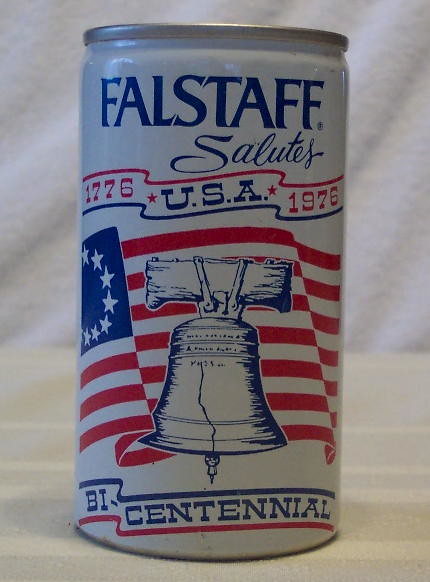This indoor photograph showcases a vintage soda can designed in a Bicentennial theme. The can is predominantly white, featuring a stylized American flag with wavy stripes that horizontally spans the middle section. Centrally overlaid on the flag is a detailed depiction of the Liberty Bell, complete with its iconic crack. Above the flag, in bold blue letters, the can is emblazoned with the text, "Falstaff Salutes 1776 USA 1976," commemorating the 200th anniversary of the United States. The word "Bicentennial" is prominently displayed beneath the Liberty Bell. The red, white, and blue color scheme adds a patriotic flair, accentuated by the red-colored dates. This collectible can visually celebrates the spirit and history of America's founding.